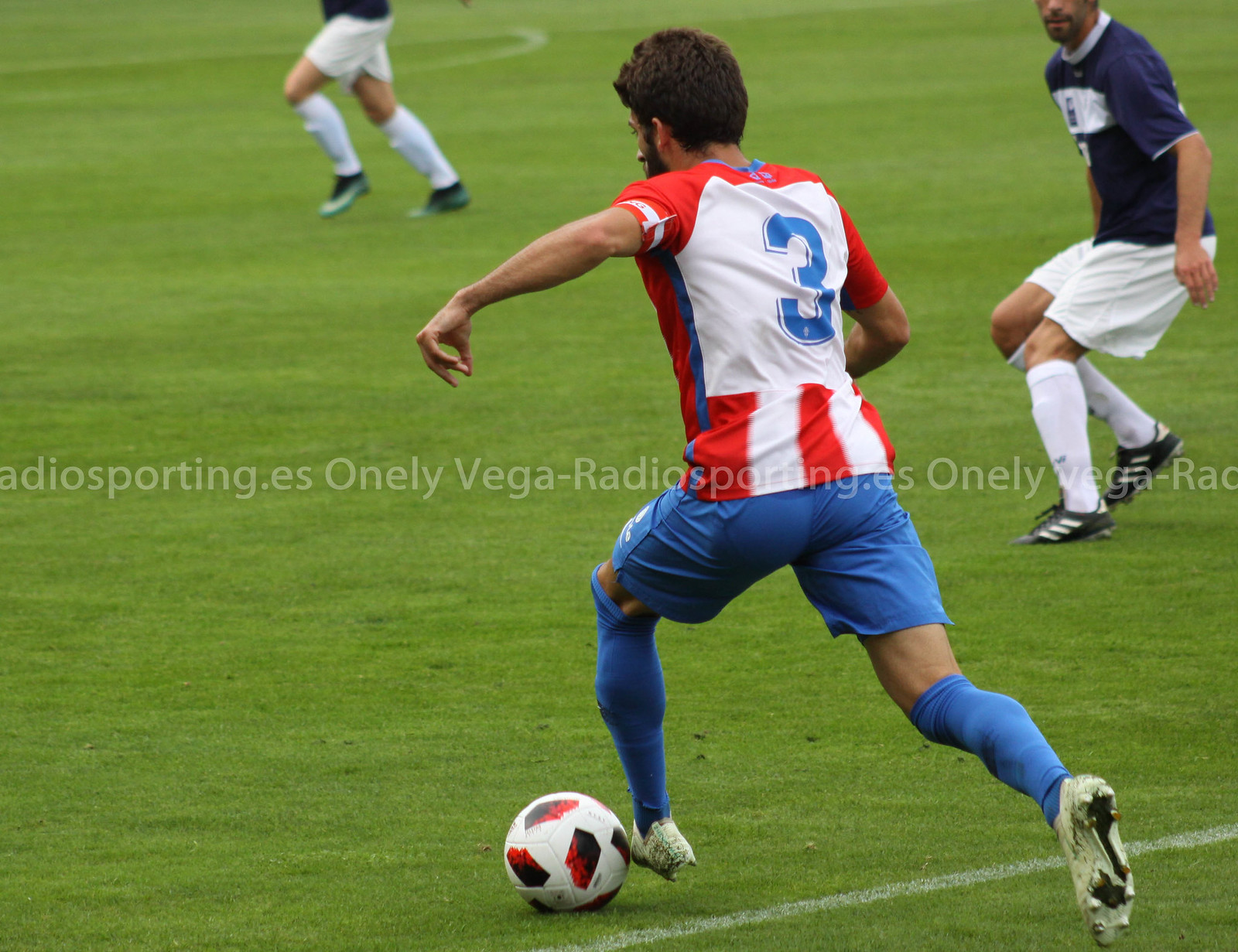This photograph captures an intense moment in a soccer match featuring three players on a green, wide soccer field. The foreground player, sporting a red and white jersey with the number three, blue shorts, blue socks, and white soccer shoes, is in motion with the soccer ball positioned near his left foot. He has brown hair and a beard, and his left arm is raised in an action pose. The soccer ball he is controlling is decorated with black and red shapes on a white background. In the top right of the image, another player is visible wearing a navy blue jersey, white shorts, white socks, and black soccer shoes with white stripes. To the top left, a third player is running, dressed in a blue shirt, white shorts, white socks, and black soccer shoes. The grassy field is marked with a clear white line running beneath the main player's feet. The detailed elements of the uniforms and their positions emphasize the dynamic nature of the game, while the background provides context to the scale and layout of the playing field.